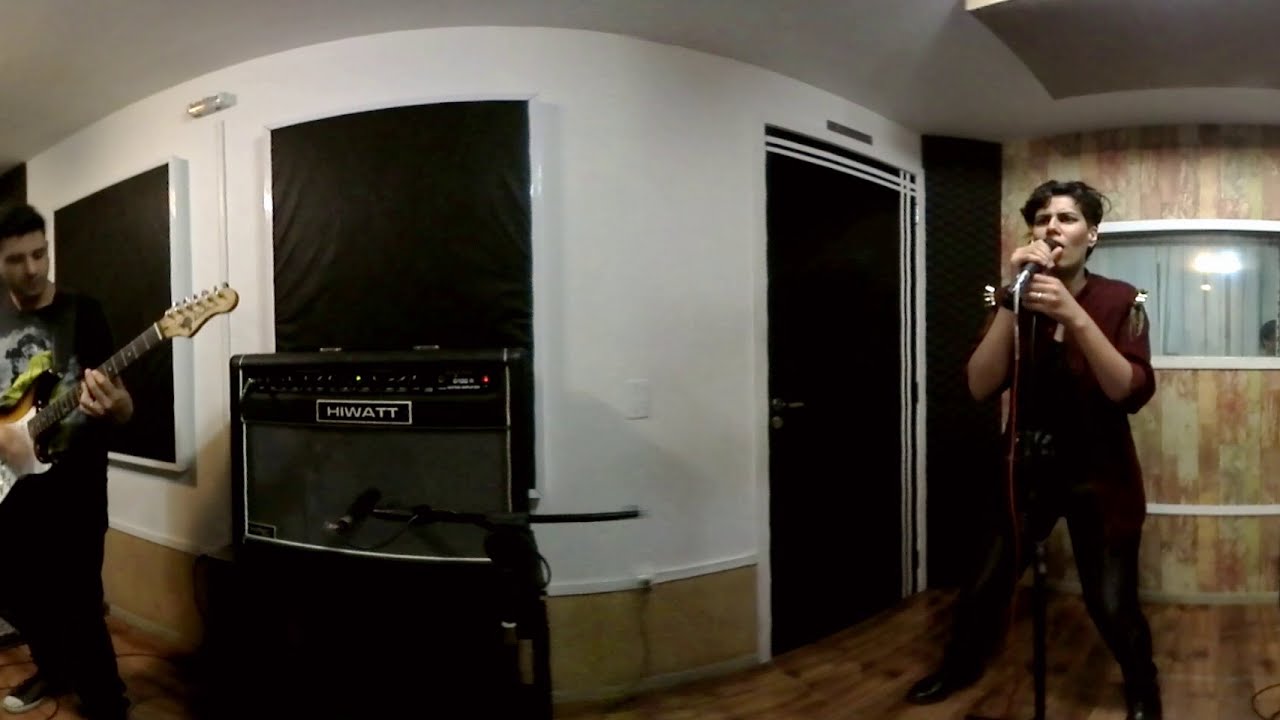In this detailed image, a young band appears to be in the midst of practice or possibly recording in a studio-like setting. The main focus is on the lead singer, a young man in his 20s with dark hair, who is intensely singing into a microphone. He is wearing a red shirt, black pants, and dress shoes. His left hand is grasping the microphone, absorbing in his performance. Adjacent to him is a guitarist, another young man dressed in a black shirt and black pants, also with dark hair. He is seen playing his guitar which is connected to a Hiwatt amplifier, identifiable by its prominent branding. The studio environment is detailed with a brown booth that has a window adorned with white curtains behind the singer. To the left, there is a larger booth area featuring a curved black door and two black windows on its left side. A speaker, also labeled with "Hiwatt," stands in front of the first window, accompanied by a recording microphone. Although only part of the guitarist's body is visible, his fingers are actively engaged with the guitar strings. The overall setup, including scattered audio equipment and lack of visible audience, conveys a focused and immersive band practice session.